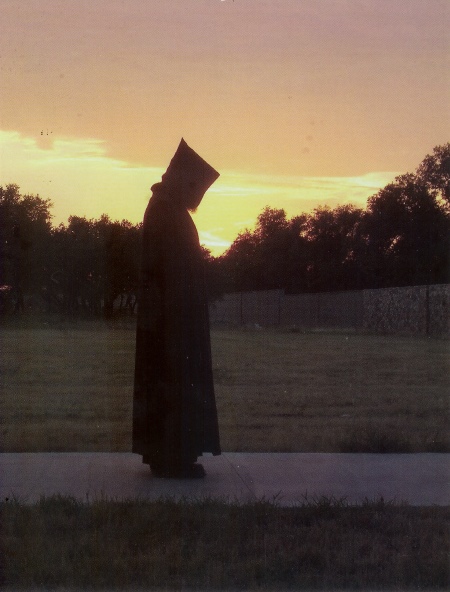This photograph captures a hooded figure standing on a concrete pathway at sunset, enveloped in a long black cloak that reaches down to their ankles. The figure's head is slightly bowed, obscured by what appears to be a hood or a bag-like covering, making it impossible to discern any facial details or even determine if it's a man or a woman. The scene is bathed in the warm, golden hues of the setting sun, casting yellow and brown tones across the sky, while some clouds are tinged with reddish-pink and yellow from the natural sunlight. 

The pathway the figure stands on cuts through a grassy area, leading towards a fence that separates the viewer from a wooded field beyond. Trees populate the background, adding depth and a sense of isolation to the scene. The overall effect is one of solitude and mystery, with the cloaked individual standing motionless amidst this serene yet slightly eerie landscape.